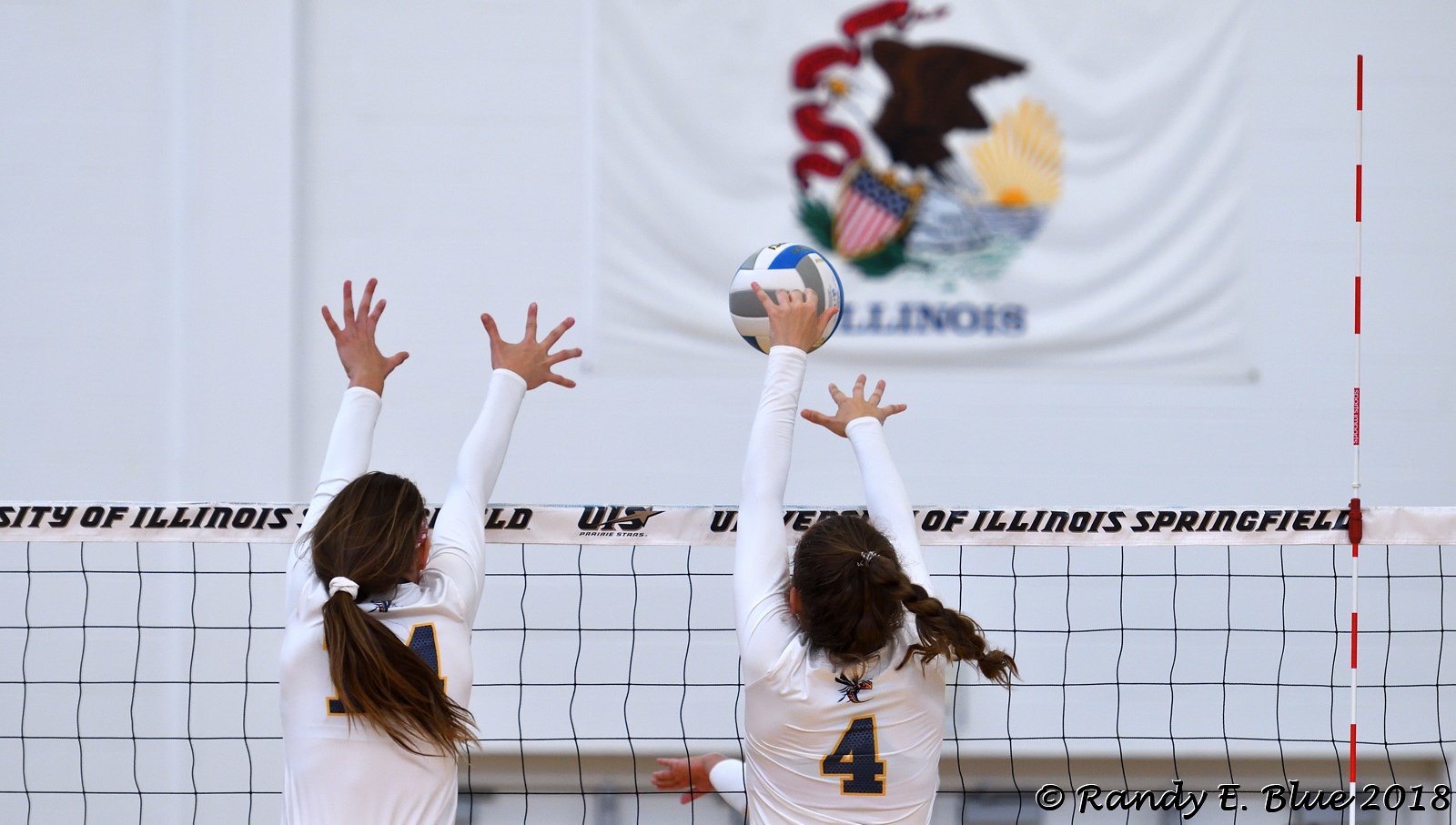In this dynamic sports photograph from a volleyball match, we see a close-up action shot at the net's right side featuring two young women in mid-air. Both are dressed in long white-sleeved jerseys with blue numbers and gold accents. The player on the left, partially obscured by her dark ponytail, is likely wearing number 14, while the player on the right, with her ponytail swung to her shoulder, clearly displays the number 4. The player numbered 4 is actively making a block against a spiked ball, supported by her teammate. The ball, seen in mid-action, is white with blue and gray segments. The net's top band is emblazoned with the words "University of Illinois Springfield," supported by a white-and-red striped rod. In the background, the Illinois state flag and a distinct banner featuring an emblem with a dark eagle and patriotic badge add depth. The image is credited to Randy E. Blue, marked "Copyright Randy E. Blue 2018" at the bottom right corner.